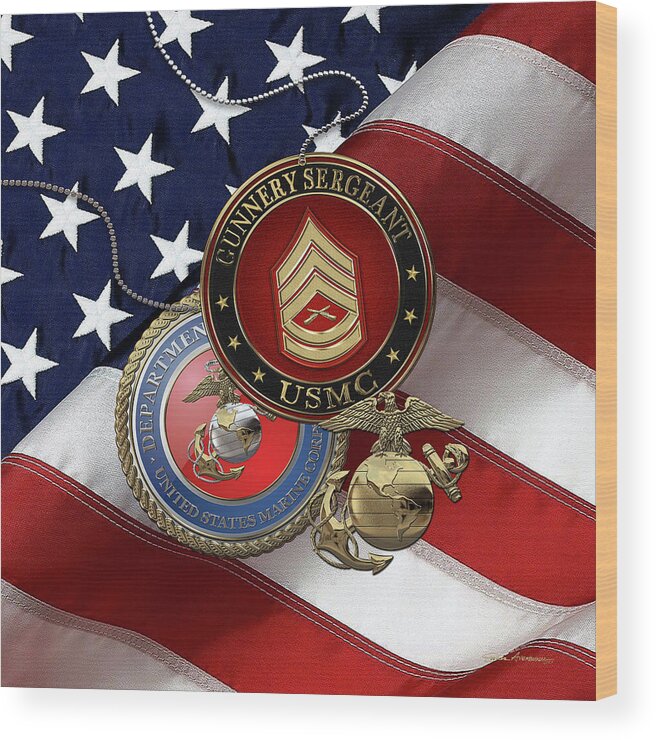This detailed image, which appears to be either a photograph or an illustration, showcases a folded American flag as the backdrop. The flag is partially spread out, displaying the blue field with white stars in the upper left corner and the red and white stripes covering the lower half diagonally. At the center, there are two prominent, oval-shaped medals. One medal features the inscription "Gunnery Sergeant USMC," flanked by three stars on each side. Another medal, partially obscured, bears the inscription "Department of the United States Marine Corps" and "Department of Defense." A smaller, bronze medal, positioned towards the bottom right, depicts a gold eagle with its wings spread, perched atop a globe, with an anchor behind it. The intricate details and the distinct military symbols emphasize the honor and significance of the Marine Corps.